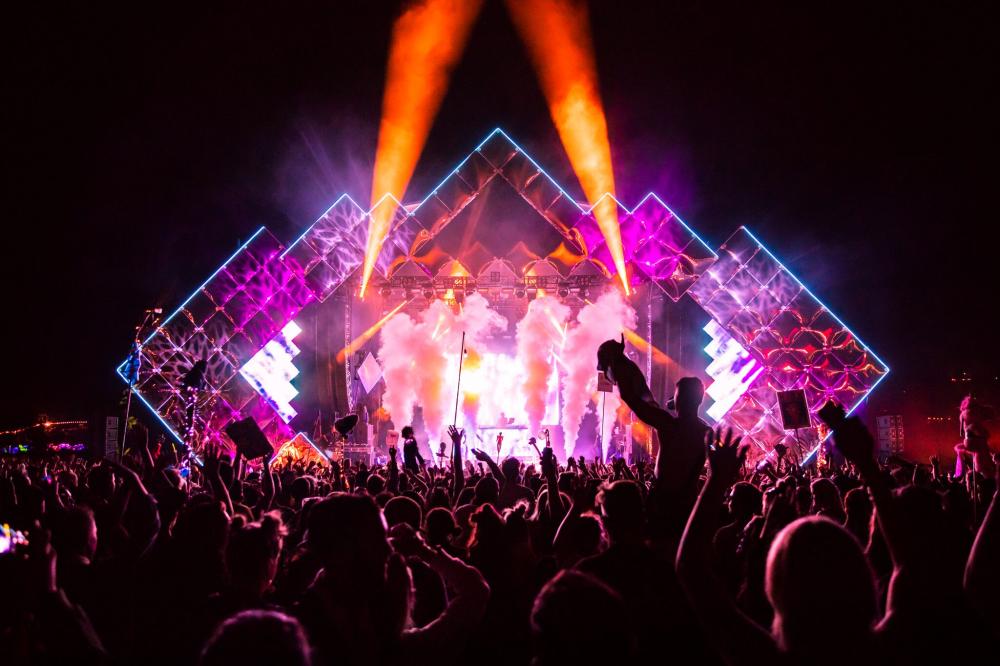The image depicts a lively 1980s rock concert set outdoors at night, with a massive crowd in attendance. The backdrop features a vivid hot pink sky and a geometric stage design characterized by a series of stacked right-angled squares and triangles, outlined in bright neon blue. The stage is illuminated with angular white-hot lights and vibrant orange spotlights flaring upward. Six columns of smoke, three on each side, shoot up from the stage, adding to the dramatic atmosphere. The stage decorations include purple translucent tiles lit up in various shades of pink and orange. The crowd, visible primarily as silhouettes outlined in the pink light, is animated with arms raised, some people perched on others' shoulders, and a few possibly holding up cell phones or posters. The entire scene is framed by a stark black border, making it hard to distinguish finer details of the audience and performers, but capturing the essence of an electric and immersive concert experience.